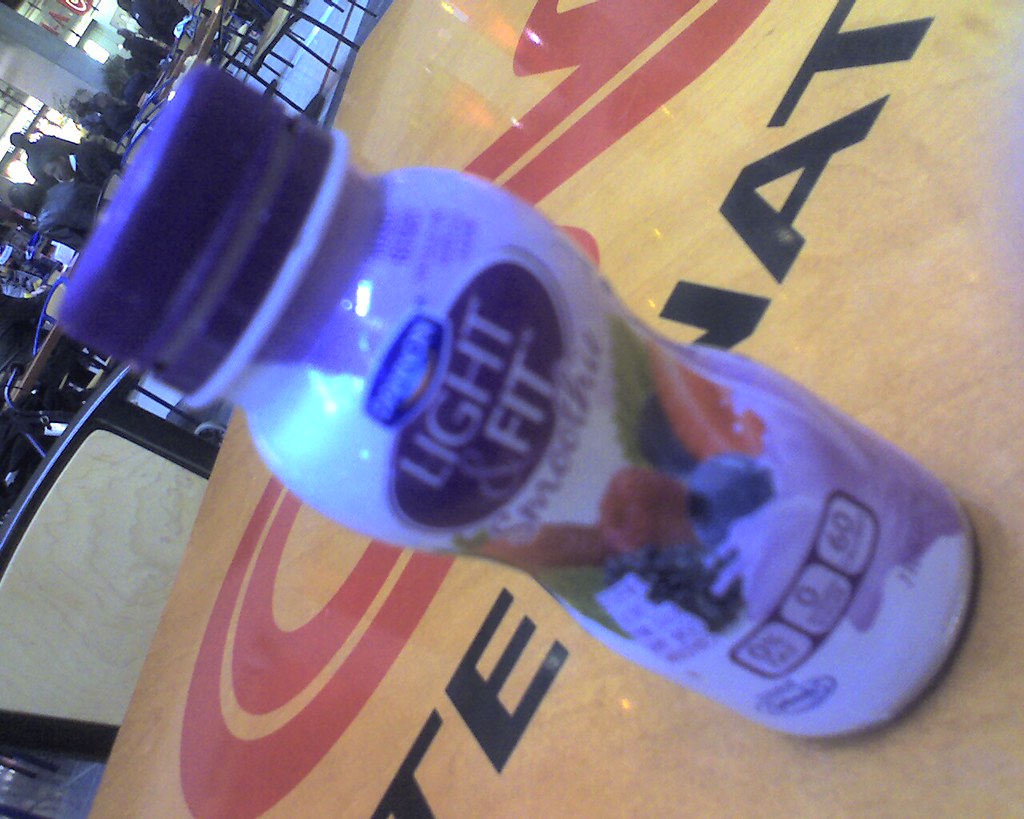The image features a close-up of a slightly tilted Light & Fit Smoothie container resting on a brownish table. The container is somewhat out of focus, making it challenging to discern details clearly. The label indicates it is a Dannon product, although the brand name is blurry. Prominently displayed on the label is the "Light & Fit Smoothie" logo, accompanied by realistic images of raspberries, strawberries, and blueberries transitioning into a liquid form. The bottom portion of the label shows some numbers, presumably indicating the caloric content. The container is capped with a distinctive blue lid. In the background, which is clearer than the foreground, several people are seated at tables in what appears to be a cafeteria or a mall food court setting, specifically noticeable in the top left-hand corner of the image.